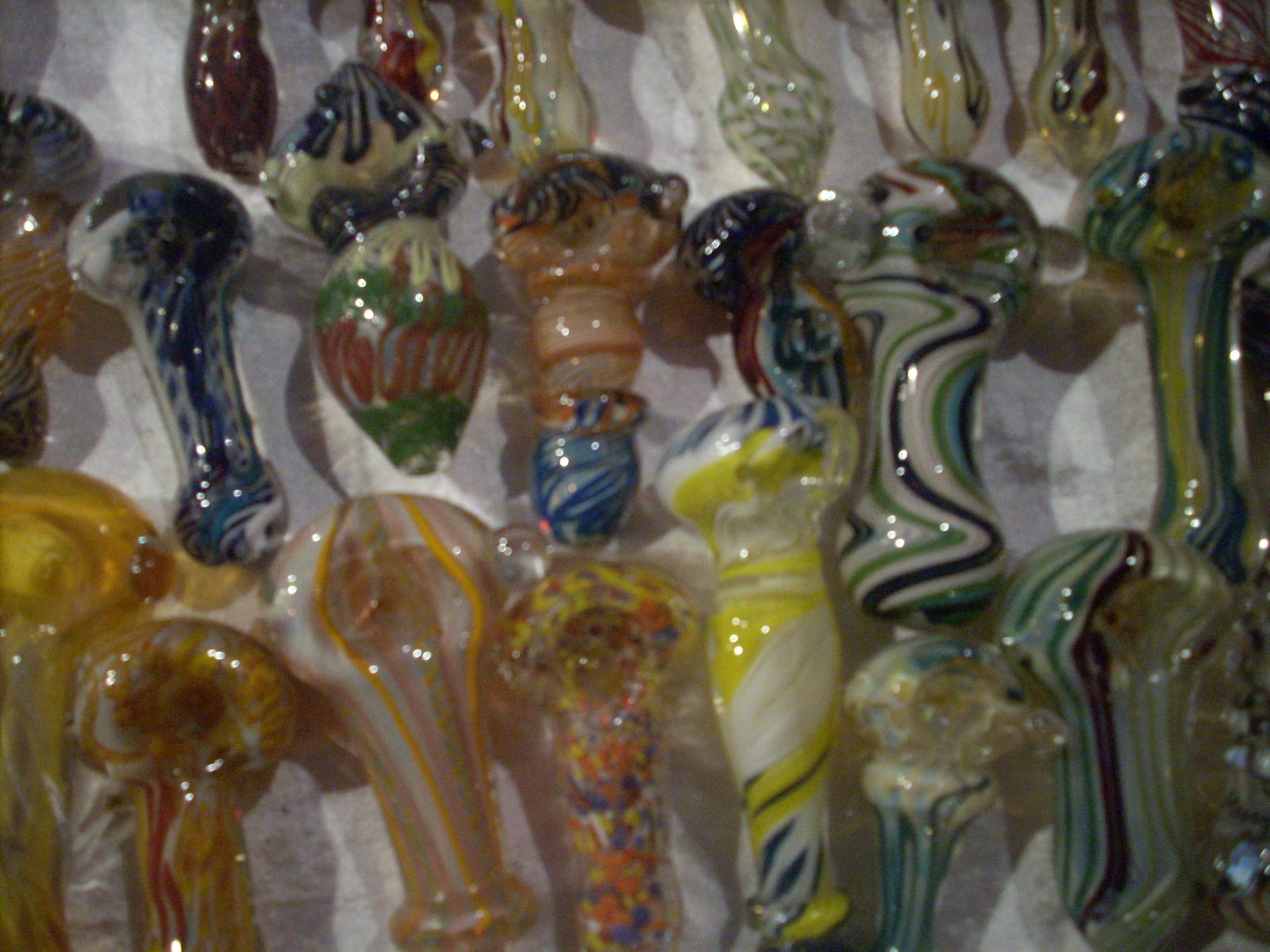This photograph features an array of intricately detailed glass pipes, meticulously laid out on a white background, likely a cloth or sheet. The collection consists of approximately 20 pipes, showcasing a diverse range of shapes and sizes. Some pipes have rounded tops with elongated bottoms, while others exhibit corkscrew-like middles. The glass pipes vary in color and pattern; several feature vivid multicolored stripes or wavy designs, while others are solid in color. Centered in the image is a particularly striking pipe characterized by a greenish background adorned with dark blue and green stripes. Other notables include a pipe with a vibrant yellow and white palette, blue and green striped pipes, and complex patterns involving colors such as navy blue, orange, yellow, and red. The pipes are arranged in three rows, with some overlapping, casting distinct shadows on the white backdrop. Despite the image being somewhat dark and slightly blurry, the elaborate patterns and vivid colors of the glass pipes are clearly visible.